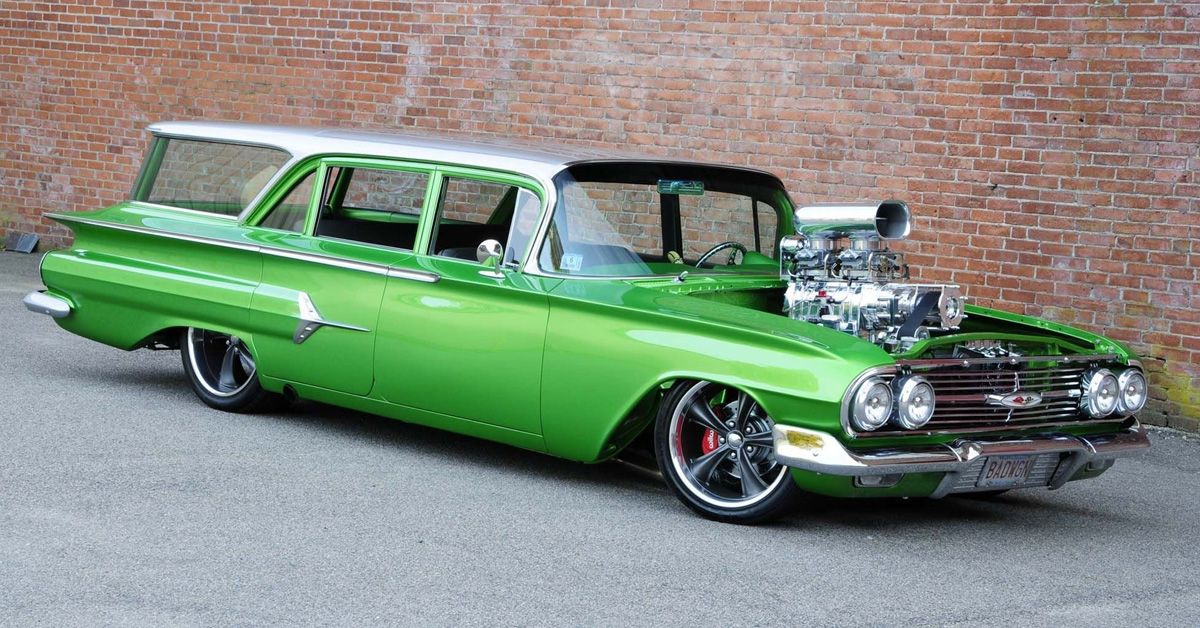The image features a striking, bright green, classic Chevrolet car parked on a gray paved street or alley, in front of a red brick wall which runs diagonally from the top left to the right and diminishes in height towards the right. The elongated vehicle has a glossy, metallic finish and a distinctively sleek design, characterized by its two side windows and a large clear back window. Its eye-catching front displays an exposed engine which rises prominently in front of the windshield, adorned with a large, chrome, exhaust-like cylinder that resembles a cannon. This feature adds a unique, almost fantastical element to the car. The roof of the vehicle glistens with a silver hue, complementing its vibrant green body. The license plate reads "Bad Wagon," hinting at the car's special, possibly custom, nature.